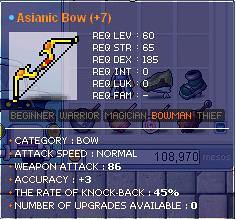The image is a detailed screenshot from a pixelated role-playing game (RPG) with a bluish-toned background, featuring an inventory grid overlaid with text and graphics. Central to the image is an 8-bit pixelated graphic of a yellow bow within a white square, labeled at the top in orange text: "Asiatic Bow +7". The text next to the graphic provides various stats and requirements, abbreviated or fully written, including: 

- Required level: 60
- Required strength: 65
- Required dexterity: 185
- Required intelligence: 0
- Required luck: 0
- Required fame: beginner, warrior, magician, bowman, thief

Additional details include:

- Category: Bow
- Attack speed: Normal
- Weapon attack: 86
- Accuracy: +3
- Knockback rate: 45%
- Number of upgrades available: 0

The background of the image includes a grid pattern suggestive of an inventory system, with some cells filled, and a brick pattern beneath. It also appears to show game currency. The overall scene portrays a typical user interface from a retro-style RPG game.